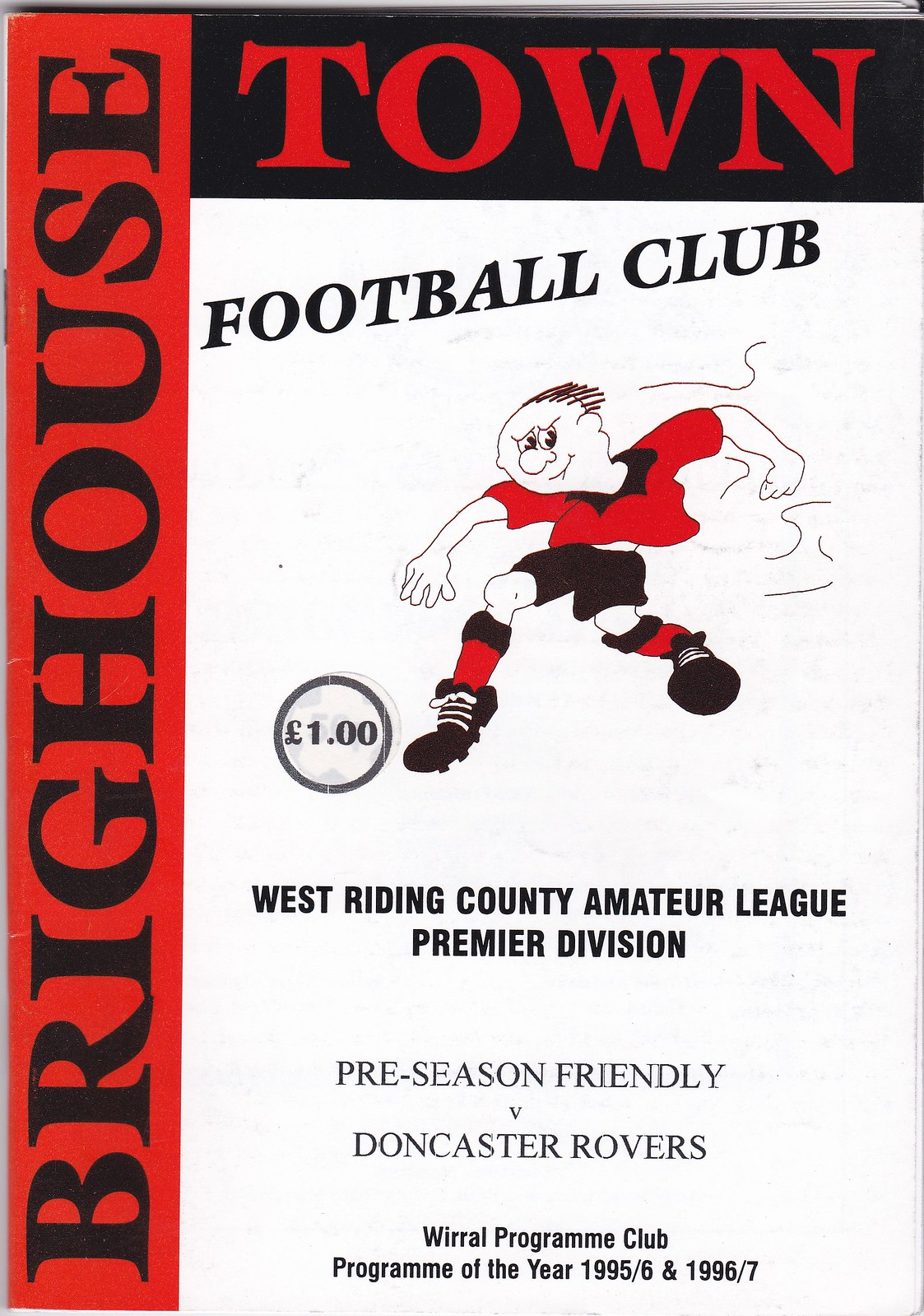The front page of a magazine features a striking design on a white background. A vertical red rectangle runs up the left side with the words "Brick House" typed in black block font, oriented sideways. On the top of the page, a black rectangle contains the word "Town" in red font. Below this, the text "Football Club" is written at a slightly slanted angle. The center of the page showcases a cartoon image of a male soccer player in action, wearing a red jersey, black shorts, red socks, and black sneakers, possibly running or kicking a ball. To the right of the player, a circle displays "one euro" inside it. Further below, the text reads: 

West Riding County Amateur League
Premier Division
Preseason Friendly vs. Doncaster Rovers

The bottom of the page highlights accolades, stating: 

World Program Club, Program of the Year 1995-96 and 1996-97.